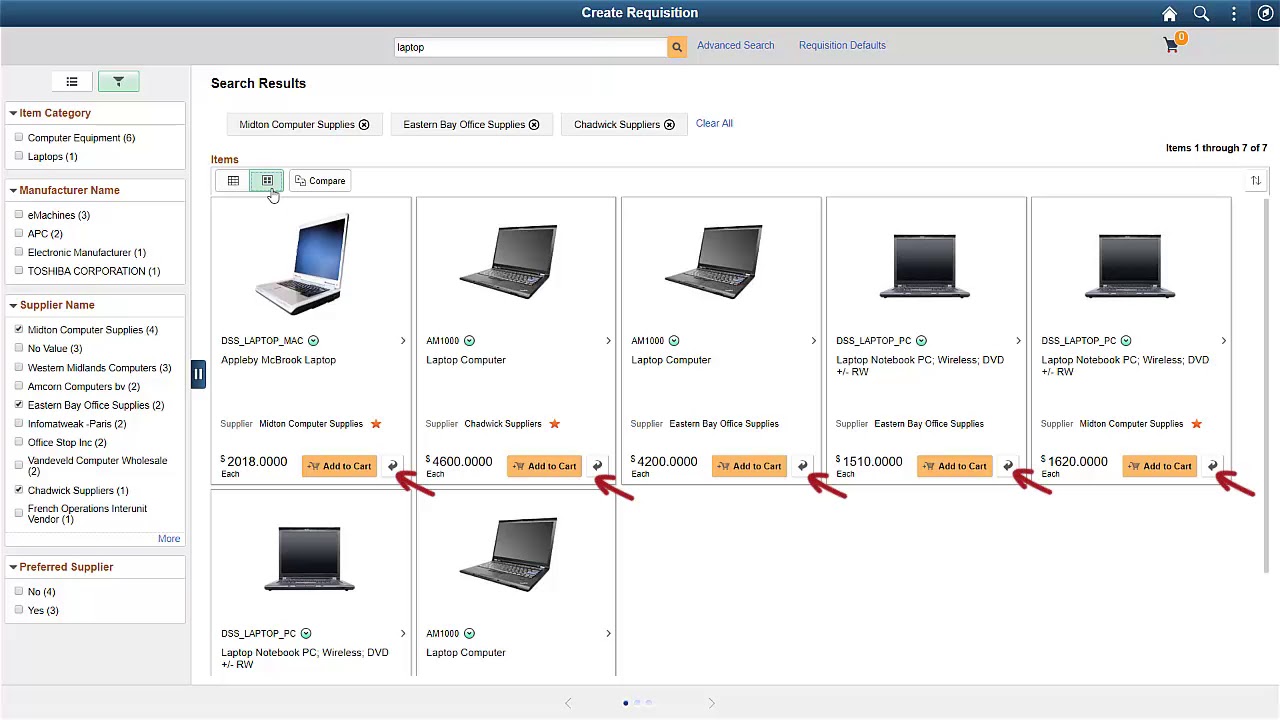This image depicts a website interface titled "Create Requisition" at the top, highlighted in a blue bar with white text. To the right of the title, there is a home icon, a search bar, and a vertical ellipsis (three vertical dots). 

Below the blue bar, a grey section contains a central search bar with the placeholder text "laptop" accompanied by an orange magnifying glass icon on the right. This section also features two blue options for "Advanced Search" and "Requisition Defaults."

The main page is split into two sections. On the left side, a menu starts with the header "Item Category" in red. Below are two entries: "Computer Equipment (8)" and "Laptops (1)," where the numbers in parentheses indicate the count of items. Next, the menu lists "Manufacturer Name" in red, displaying potential manufacturers with checkboxes next to each, all currently unchecked. They include: 
- eMachines (20) 
- APC (2) 
- Dektonic Manufacturer (1)
- Toshiba Corporation (1)

The "Supplier Name" section follows, enumerating suppliers and their item counts, some with checkmarks:
- Edison Computer Supplies (4) - checked
- No Value (2)
- Western Midlands Computers (3)
- Amcon Computers (2)
- Eastern Bay Office Supplies (2) - checked
- Informer Work Pass (2)
- Office Lab Inc. (2)
- Vanderfield Computer Wholesale (2)
- Chadwick Supplies (2)
- French Operation Internet Vendor (1)

Next is "Preferred Supplier," indicating "No" (4) and "Yes" (3) options.

The right section showcases search results with three tags labeled "Modern Computer Supplies," "Eastern Bay Office Supplies," and "Chadwick Supplies," along with a blue "Clear All" button. This section displays a grid of five laptop images in the first row, four black and one silver, all open. 

The laptops have blurry descriptions with the following details visible:
- The silver laptop has a blue screen with text: "D88_laptop MAC," priced at $2018,000, and features a red "Add to Cart" button.
- The next two are black laptops labeled "AV100," priced at $4800 and $4200, respectively.
- Two more laptops are labeled "D88_laptop_PC" priced at $1610 and $1620.

The second row features additional laptops of the same kind, though their prices are cut off in the image.